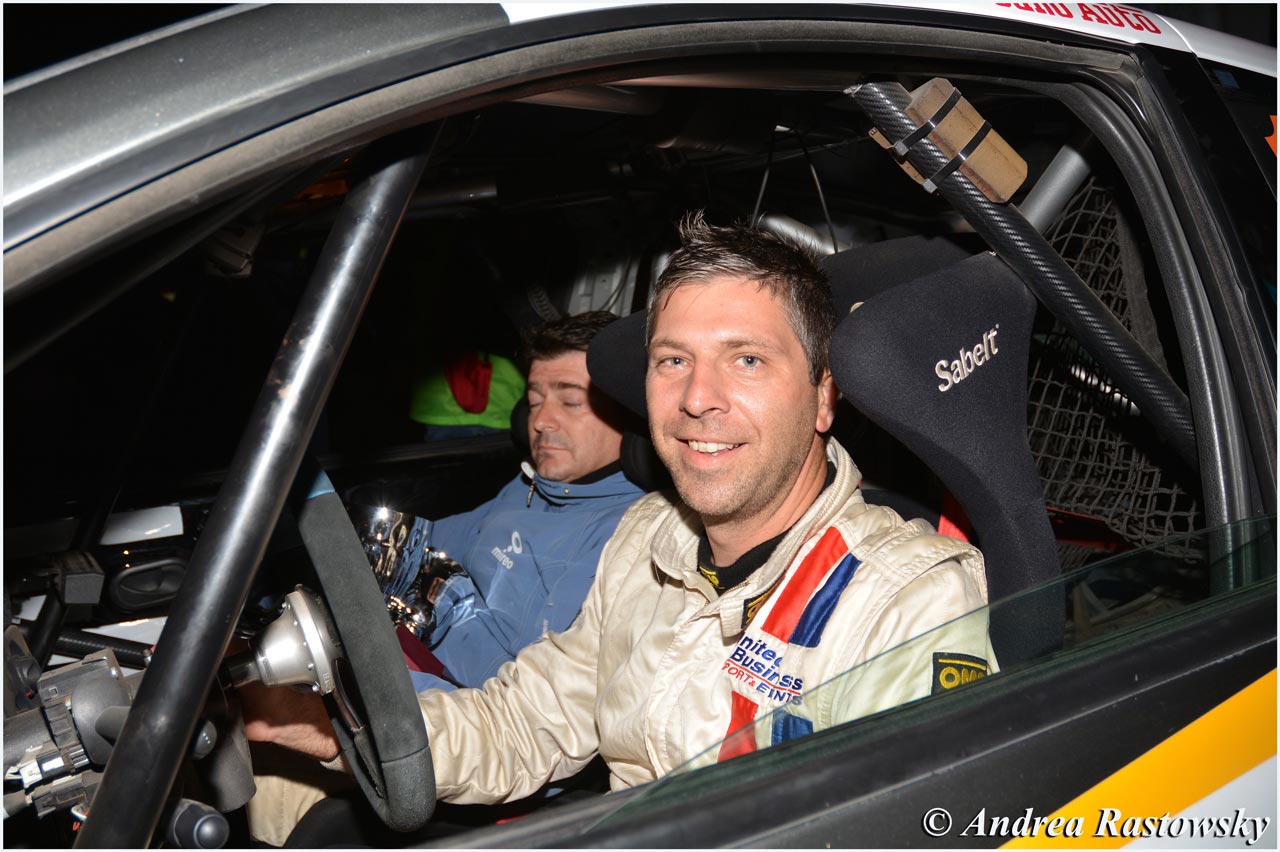This copyrighted photograph by Andrea Ratowski captures a detailed and dynamic scene of a race car driver and his passenger. The driver, a middle-aged white man with short brown hair, is seated in the driver's seat of a race car. He is wearing a white racing uniform adorned with red and blue stripes and a sponsor logo on his left chest that reads "United Business." Visibly delighted, he smiles warmly at the camera, his hand resting on the steering wheel. 

The car, viewed primarily from the side through the front driver's window, reveals intricate details like the roll bar and harnesses designed to protect the driver’s head and neck. Adjacent to him in the passenger seat is another man dressed in a blue pullover sweatshirt, sporting short black hair. His eyes are closed, giving the impression that he might be asleep or was caught mid-blink. He holds a silver trophy, suggesting a celebratory moment following a race.

Even the background elements such as the top of the car and the driver’s door panel are subtly included in the frame, enhancing the completeness of the scene. Finally, in the bottom right corner, the name Andrea Ratowski is imprinted in white, marking the photograph's artistic ownership.